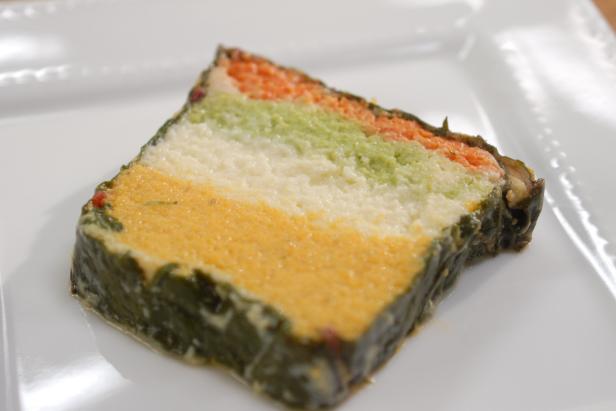This is a detailed color photograph captured in landscape mode, featuring a close-up view of a layered food item set on a square white plate, visible only in portions without showing its edges. The image showcases a roughly square piece of food positioned diagonally on the plate, with white space surrounding it on all four sides. The slice consists of four distinct layers: from bottom to top, there is a large reddish-orange layer resembling tomato, followed by a greenish stripe that could be avocado or guacamole, then a white or cream-colored layer suggestive of cream cheese, and topped with a small orange layer, possibly reminiscent of cheddar cheese. The entire piece is surrounded by a brownish-green coating, which could be herbs or spinach. The food's consistency appears to be somewhat mushy or pureed, similar to mashed potatoes, and it may be a vegetable-based dish. The foreground of the photograph is slightly blurred, drawing more attention to the layers and texture of the presented slice.